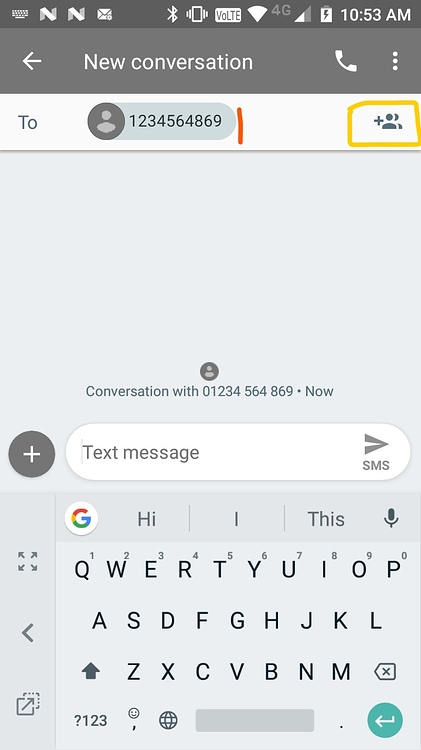The image depicts an individual texting on a cell phone with unusual proportions, being taller but not as narrow as modern smartphones. The background is a pale gray. The top section of the screen features three horizontal rectangles: the first one displays various standard cell phone information such as signal strength, battery life, 4G connectivity (indicating the era before the widespread adoption of 5G), and the current time, which is 10:53 a.m.

The interface is in "New Conversation" mode with a generic profile placeholder image and numbers "1234 564 869" indicating the recipient. There's an "Add New Person" icon highlighted in yellow in the upper right corner. The middle of the screen repeats the recipient's number, clearly preparing for a message composition. At the bottom of the screen, there is a text input field labeled "Text Message." The cell phone keyboard layout is shown here, with numbers 1 through 9 presented in superscript above the respective letters.